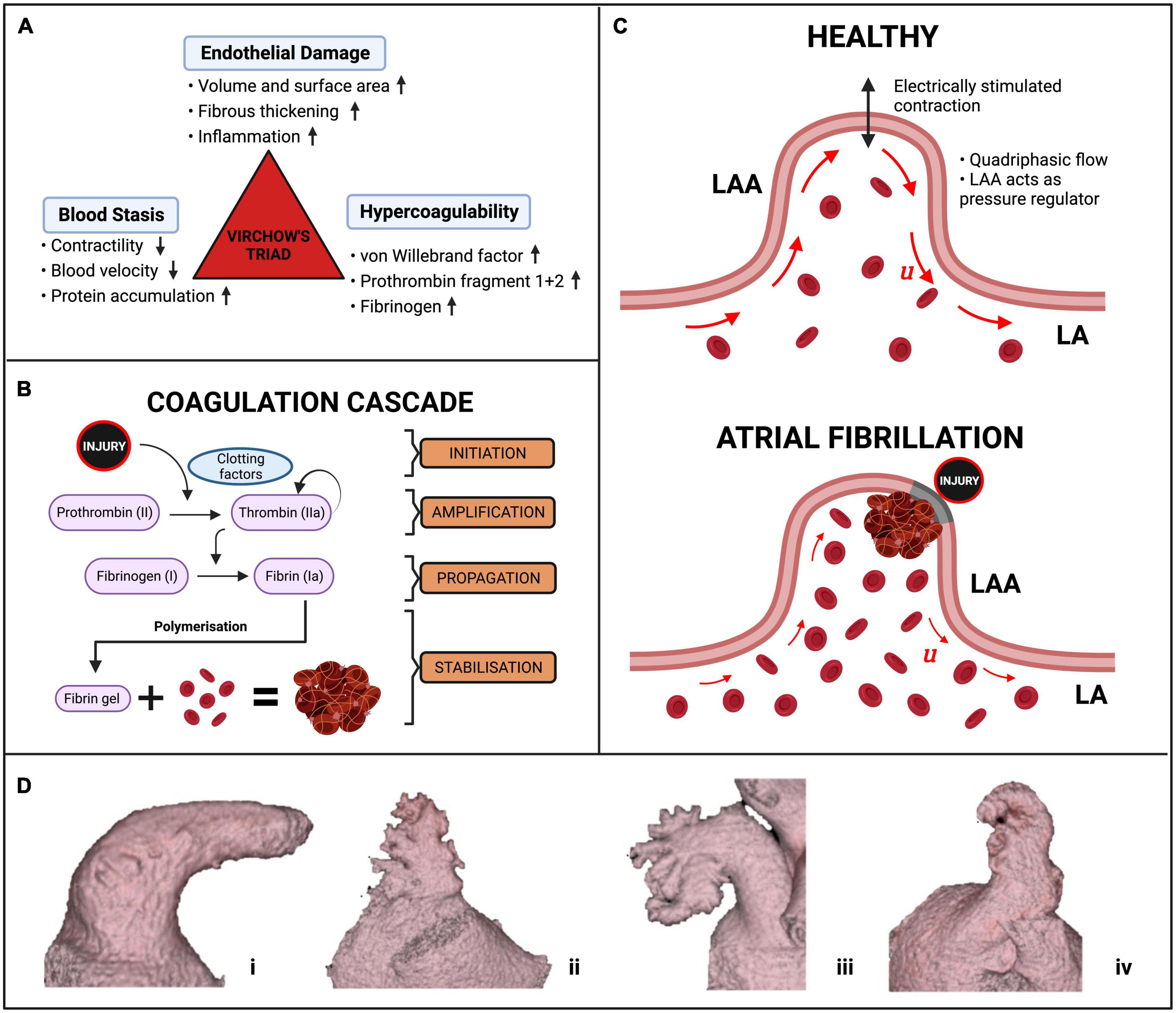This detailed infographic on heart health is divided into four labeled sections (A, B, C, and D) and is designed to educate about various aspects of cardiovascular conditions.

**Section A: Virchow's Triad**  
A large red triangle in the center features the heading "Virchow's Triad," highlighting the three main factors contributing to thrombosis: **Endothelial Damage**, **Blood Stasis**, and **Hypercoagulability**.  
- **Endothelial Damage** is in a rectangle with bullet points below: "Volume and Surface Area," "Fibrous Thickening," and "Inflammation," each marked with an upward arrow.
- **Blood Stasis** is indicated at the bottom right of the triangle with bullet points: "Contractility" and "Blood Velocity," both with downward arrows, and "Protein Accumulation" with an upward arrow.
- **Hypercoagulability** on the left side lists bullet points: "Von Willebrand Factor," "Prothrombin Fragment 1+2," and "Fibrinogen," all with upward arrows.

**Section B: Coagulation Cascade**  
This diagram details the process of blood clot formation starting from an injury.  
- **Injury** is depicted with a black circle leading to a blue oval labeled "Clotting Factors."  
- Arrows guide to four purple boxes labeled sequentially: "Prothrombin," "Thrombin," "Fibrinogen," and "Fibrin," illustrating the pathway.  
- A black line and arrow descend to the terms "Polymerization" and "Fibrin gel + Red Blood Cells = Clot," with an annotation hinting at the end product being a clot, despite minor ambiguity in illustration.
- On the left, orange text outlines the stages: "Initiation," "Amplification," "Propagation," and "Stabilization."

**Section C: Healthy vs Atrial Fibrillation**  
This section contrasts a healthy artery with one affected by atrial fibrillation.
- The **Healthy** artery illustration shows red blood cells in circulation with annotations like "Electrically Stimulated Contraction," "Quadriphasic Flow," and notes that the "LAA" (likely referring to the left atrial appendage) acts as a pressure regulator.
- The **Atrial Fibrillation** image shows a blood vessel with labeled injury points and disrupted blood flow pathways, indicating clot formation and an irregular arrangement of red blood cells.

**Section D: Heart Condition Renderings**  
This final section provides 3D renderings of different types of cardiac or vascular damage. Detailed captions label four separate images to likely represent different stages or aspects of heart disease or injury, denoted as I, II, III, and IV in Roman numerals, showing various textures and structural differences in the heart tissue.

Overall, the infographic comprehensively illustrates crucial elements of heart health, particularly focusing on thrombosis, the coagulation cascade, arterial conditions, and visual representations of heart damage.